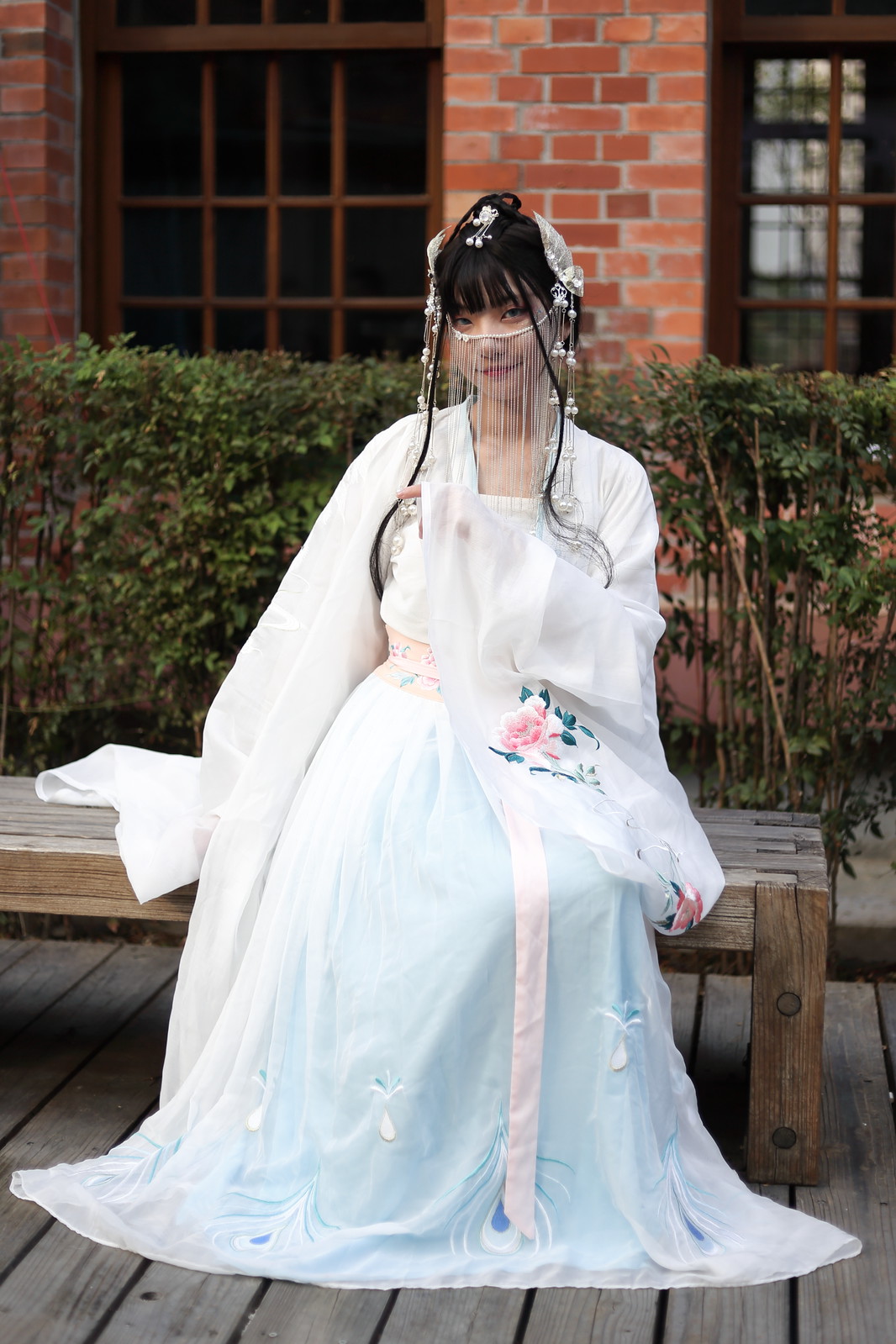The photograph captures a young Asian woman, possibly of Chinese or Korean descent, seated on a wooden bench placed on a wooden deck. She is dressed in traditional, possibly bridal, attire consisting of a long, elegant white gown adorned with pink flowers and light blue detailing near the bottom. Her hair is styled elaborately with ornaments and decorations cascading from a hairpiece, including side links of material. Notably, she wears a unique face covering, a veil made up of strings, that extends from the top of her nose down to her chest.

The setting includes green bushes directly behind her, followed by a backdrop of a brick building with large glass windows that do not reveal the inside. A door, partially visible through the glass, adds to the scene. The young woman, holding up a part of her dress with her left hand, gazes directly at the camera, creating an intimate and captivating portrait.